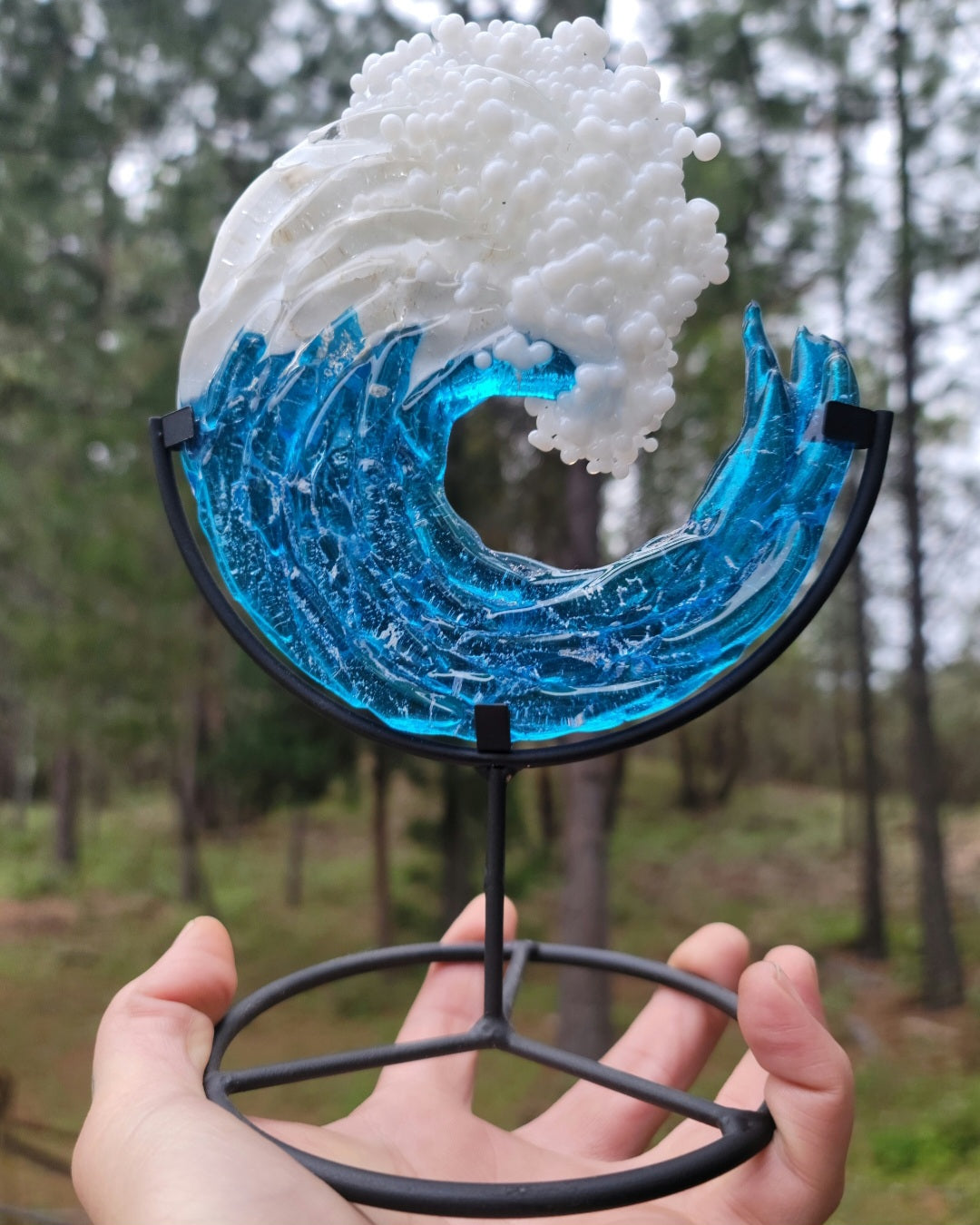A close-up image captures a person's hand holding a circular metal base, divided into thirds at the bottom. Rising from the center is a metal arch that supports a striking glass sculpture of a wave. The wave starts on the right side of the arch, with translucent blue glass swirling upward towards the left, culminating in a frothy white cap made of small, bubble-like formations. The artistic wave sits prominently in the palm of the hand, dwarfing other elements in the photo. The background reveals a blurry glimpse of tall, slender trees and a forest floor with patches of green and brown, indicating the natural outdoor setting where the photo was taken. The slightly out-of-focus trees enhance the clarity and vibrancy of the glass wave, making it the undeniable focal point of the image.